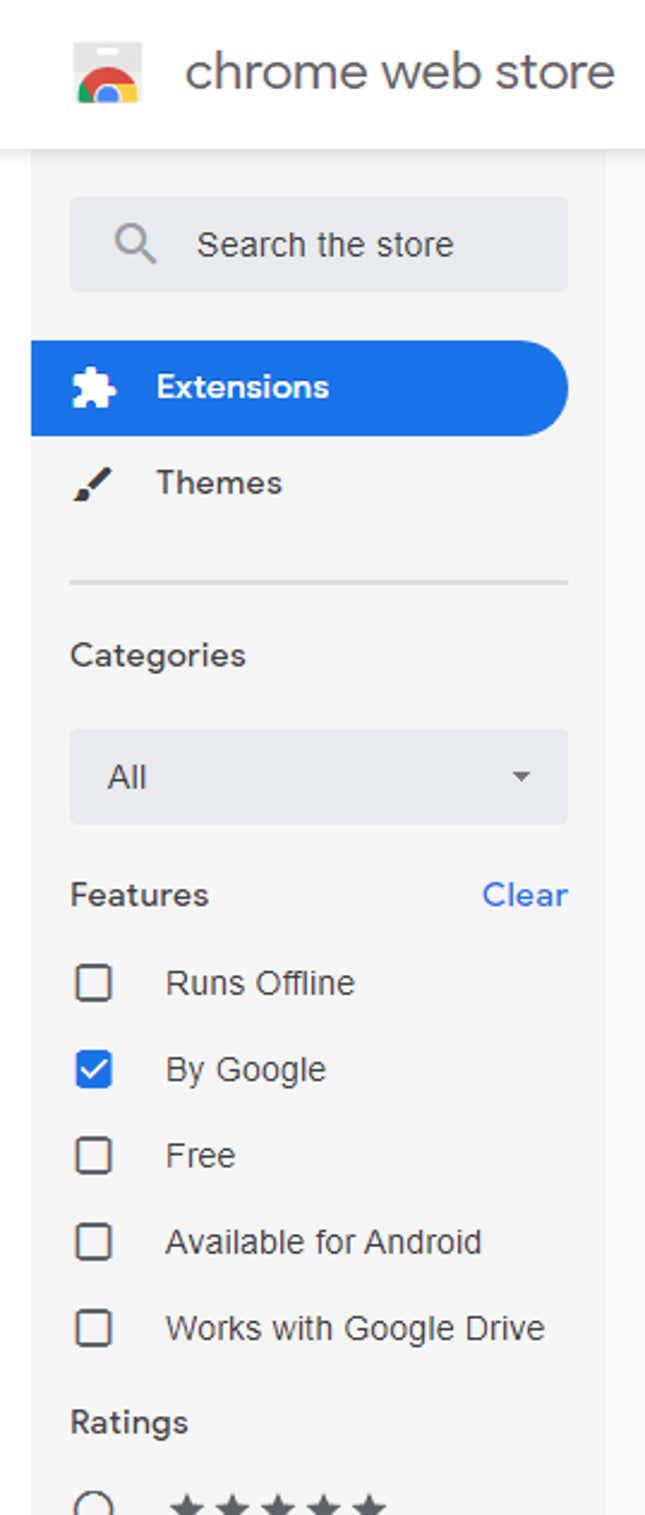The image shows the Google Chrome Web Store interface. The top portion features a white background with a partially visible Google Chrome logo displaying the characteristic green, red, yellow, and blue colors in a circular pattern. Next to the logo, in black text, is the heading "Chrome Web Store." 

Beneath this, the background transitions to gray. A gray rectangle at the top contains a gray magnifying glass icon followed by the black text "Search the Store." Towards the right, there is a partially cut-off blue oval with a white puzzle piece icon inside it and the text "Extensions" in white. 

Further down, on the left, there's a black paintbrush icon next to the black text "Themes." Underneath, there is a section titled "Categories" with a thin gray line separating it. Inside this section, a gray rectangle contains the word "All." Below, it says "Features" in black text.

On the right side, there is a blue "Clear" button. Below the "Features" heading, there are several outlined boxes with text beside each one. The second box is filled in blue and has a white checkmark, labeled "Runs Offline." The other options include "By Google," "Free," "Available for Android," and "Works with Google Drive," each with an outlined box next to them. At the bottom, there's a section labeled "Ratings," displaying five stars.